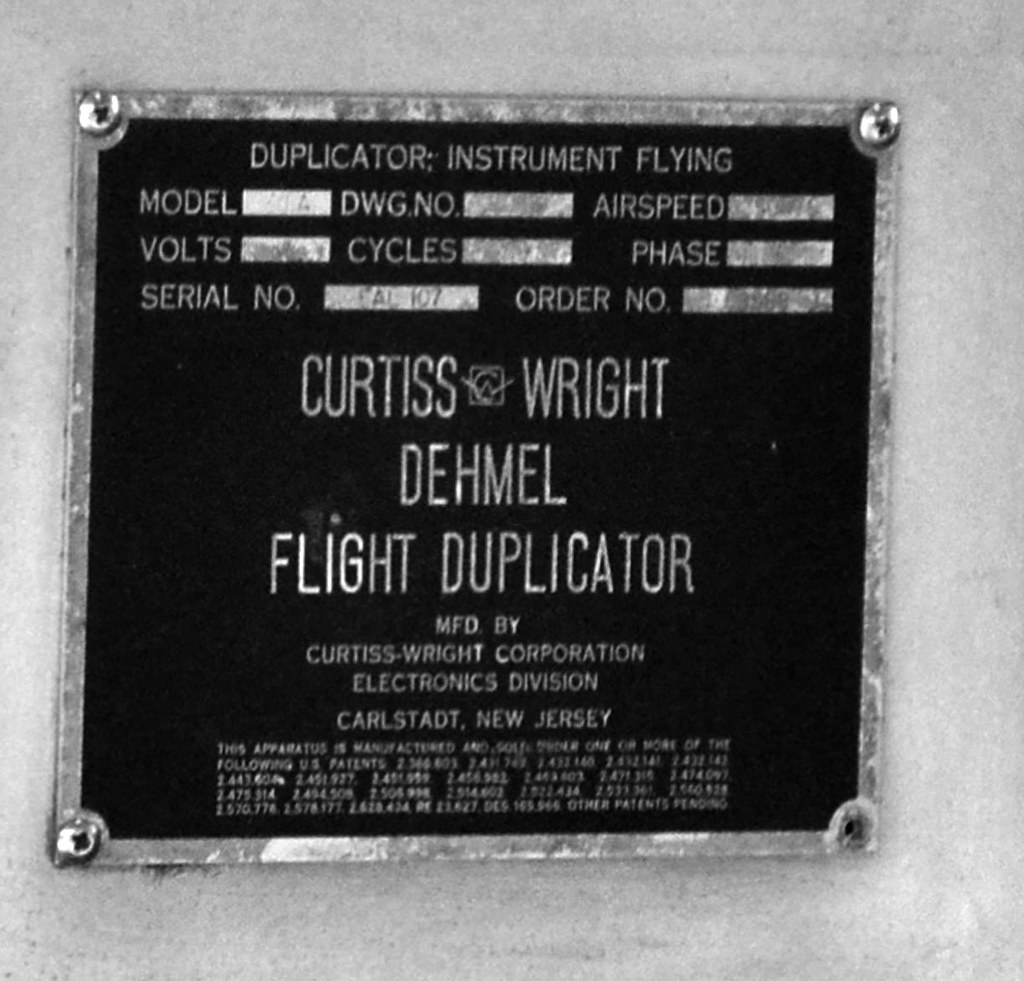This is a square-shaped metal plaque affixed with four screws, one in each corner, possibly mounted on a piece of equipment or a wall that appears to be made of stone. The plaque features a silver metal border surrounding a black background. At the top, in silver or white text, it reads "Duplicator Instrument Flying." Below this, there are several lines intended for various technical specifications such as model, DWG. NO, airspeed, volts, cycles, phase, serial number (with the visible example "AL107"), and order number, though these details are largely faded or illegible. Further down, it states "Curtis Wright Demo Flight Duplicator," followed by "MFD by Curtis Wright Corporation, Electronics Division, Carlstadt, New Jersey." In smaller text below, it mentions that the apparatus is manufactured under one or more patents, listing several patent numbers which are too small to be read clearly.